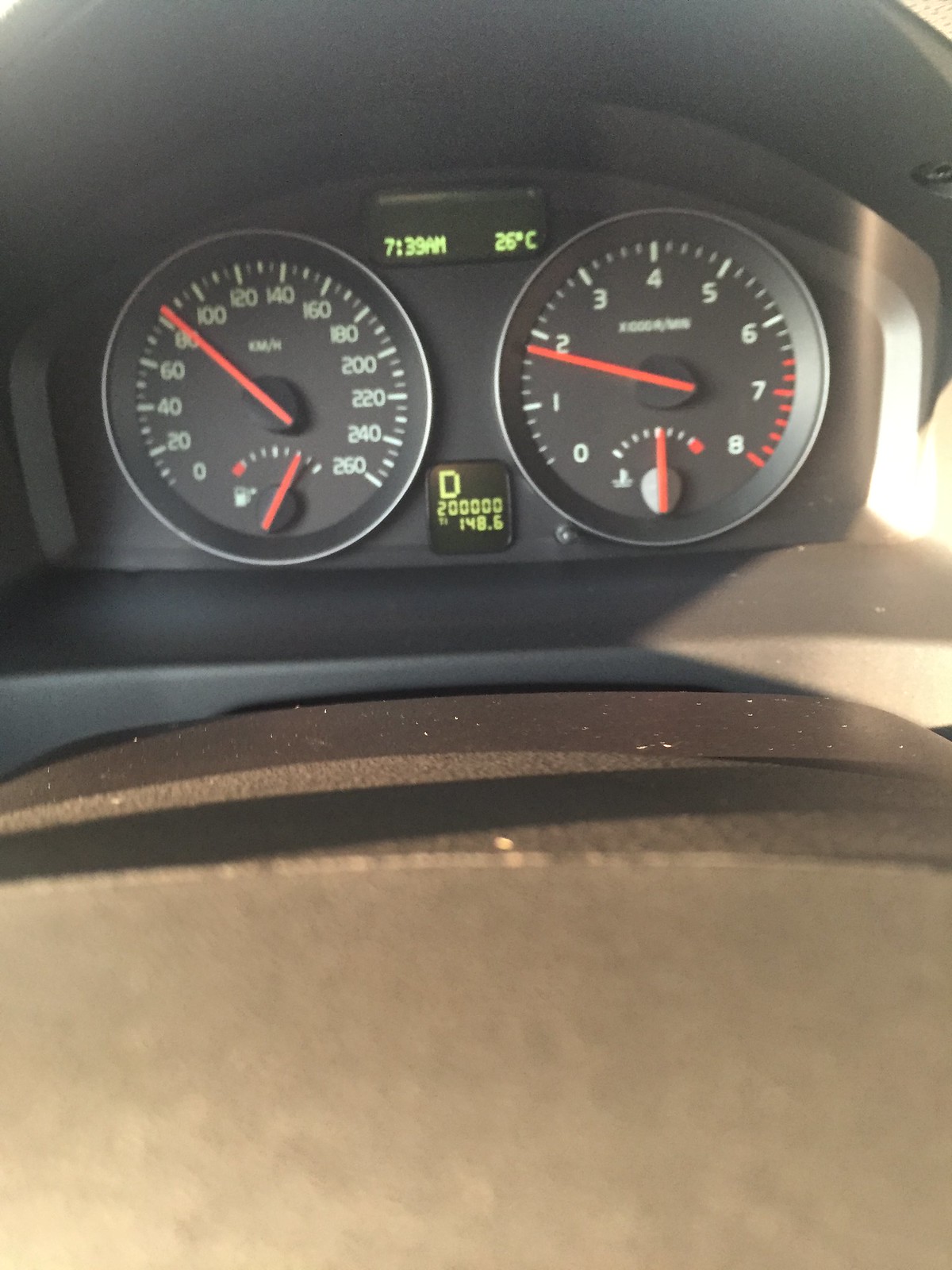This is a very tight close-up shot from the rider’s point of view of a vehicle's dashboard panel, specifically that of a bike, with part of the brown fuel tank visible in the foreground. The dashboard features two large circular dials with white numbers set against a charcoal gray background. The pointers on these dials are red. On the left is the speedometer, with its red needle pointing just above 80 kilometers per hour. Below the speedometer is a fuel gauge showing almost a full tank. On the right is the tachometer, with its needle positioned just below 2. Centered at the top of the dashboard is a digital display showing the time, 7:39 AM, and the temperature, 26 degrees Celsius. Below this display is another digital readout indicating an odometer reading of 200,148.6 kilometers.